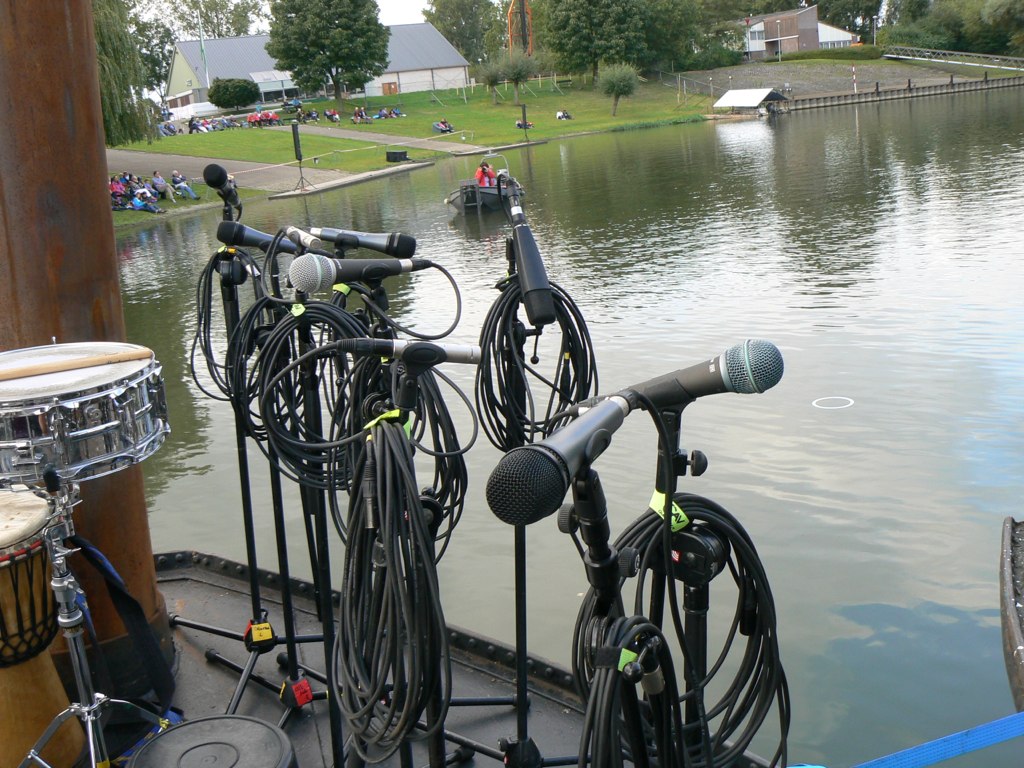The daytime color photograph captures a serene lake scene with a musical setup in the foreground, indicating preparations for a performance. The small, black stage houses several microphones on metal stands, their black cords neatly coiled and secured with Velcro ties. To the left, a snare drum with gleaming silver edges holds at least one wooden drumstick atop it.

Across the tranquil water, the far shoreline features a spacious expanse of green grass leading up to a property resembling a barn with a pitched grey roof and white walls. Scattered groups of people are seated on the bank, suggesting an audience, some perched on grassy areas, and others by a patch of brown gravel. Additionally, a lone individual in a red outfit navigates a small rowboat on the calm lake, adding to the peaceful ambiance of the scene.